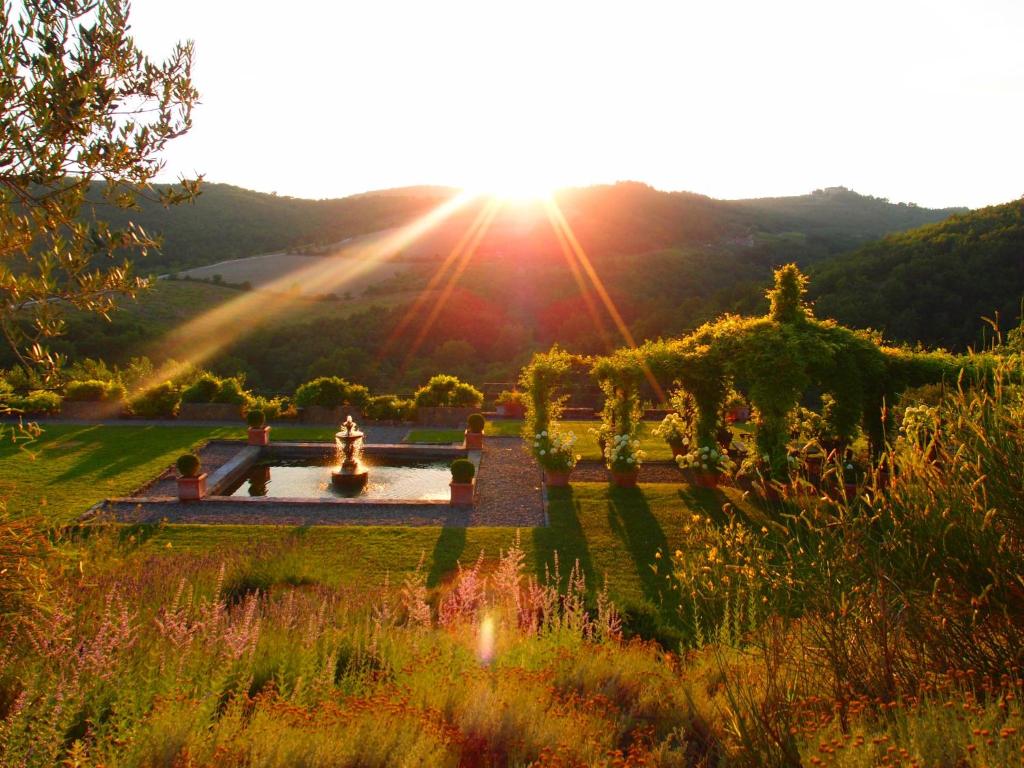The photograph captures a stunning outdoor landscape. In the distance, silhouetted against the bright, nearly white sky, is a mountain range bathed in the first light of dawn. The sun is positioned just at the top edge of the mountains, casting radiant orange and yellow rays that spread downwards and to the sides, illuminating the scene below. The middle ground features an expanse of lush greenery, with rolling hills blanketed in rich, verdant forests and grass. In the foreground, there is a meticulously landscaped garden. This garden includes an elegant square pond with a central fountain, surrounded by a brown gravel or stone walkway. Flower pots with blooming perennials and manicured greenery are thoughtfully arranged throughout the garden. To the left, a tree extends into the frame, adding a touch of natural beauty. On the right side, an arbor, covered in foliage, casts intricate shadows onto the ground, enhancing the image's depth and texture. The combination of the vibrant sky, distant mountains, and detailed garden creates a harmonious and picturesque scene.